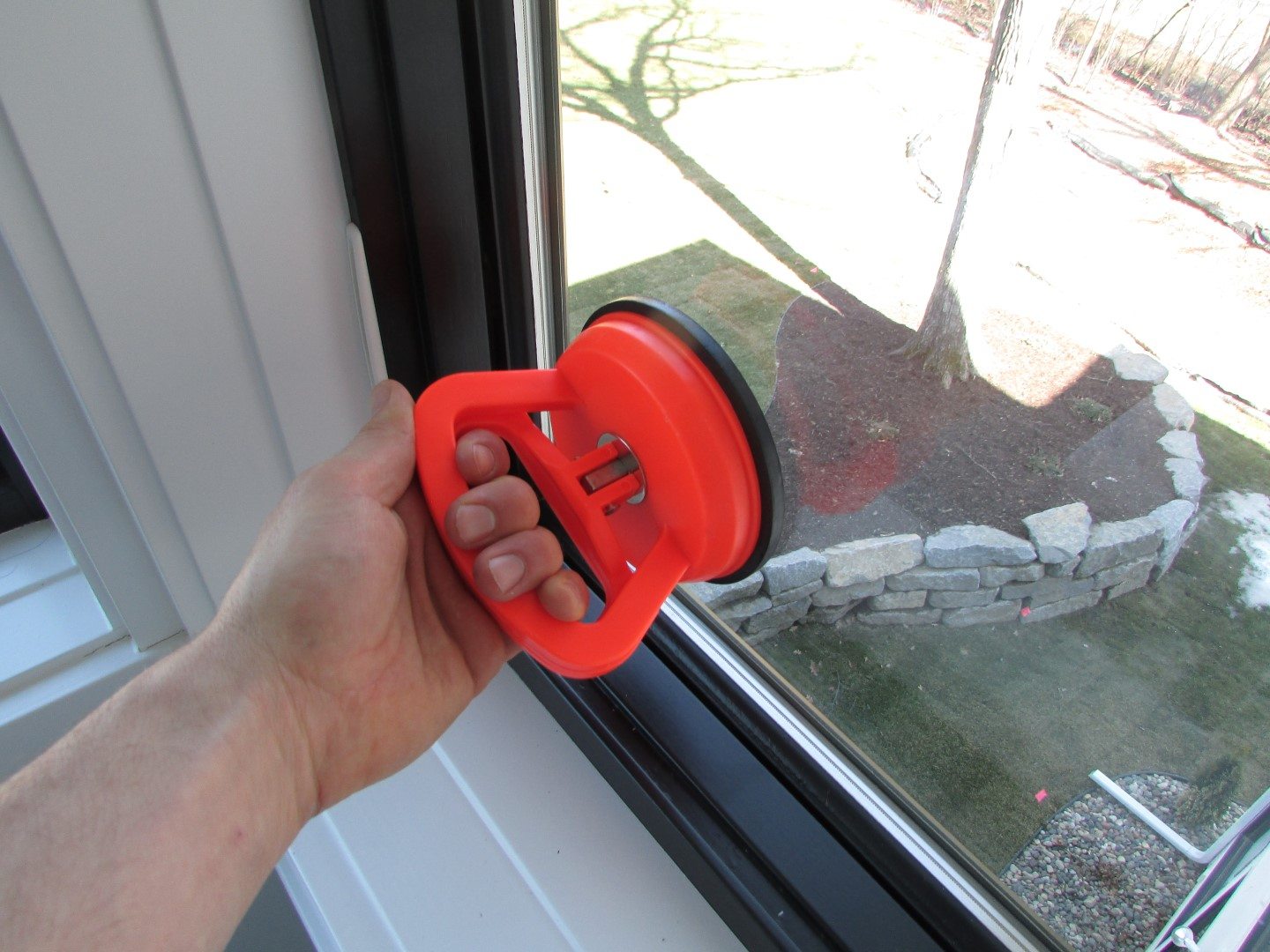A color photo captures a man's hand emerging from the bottom left, firmly gripping a bright orange suction cup tool pressed against an upstairs window. The hand, with its fingers wrapped around the handle, holds the main emphasis. The black trim of the window contrasts with the white window frame and surrounding wall. Beyond the window, you can see a small green lawn, a tree casting shadows, and brick fencing, indicating the window is on the second or third floor. The scene outside also includes a flower bed with garden stones and dark soil. The precise purpose of the tool—whether for cleaning, repairing, or another function—remains uncertain, but its prominent placement suggests it plays a critical role in the action depicted.